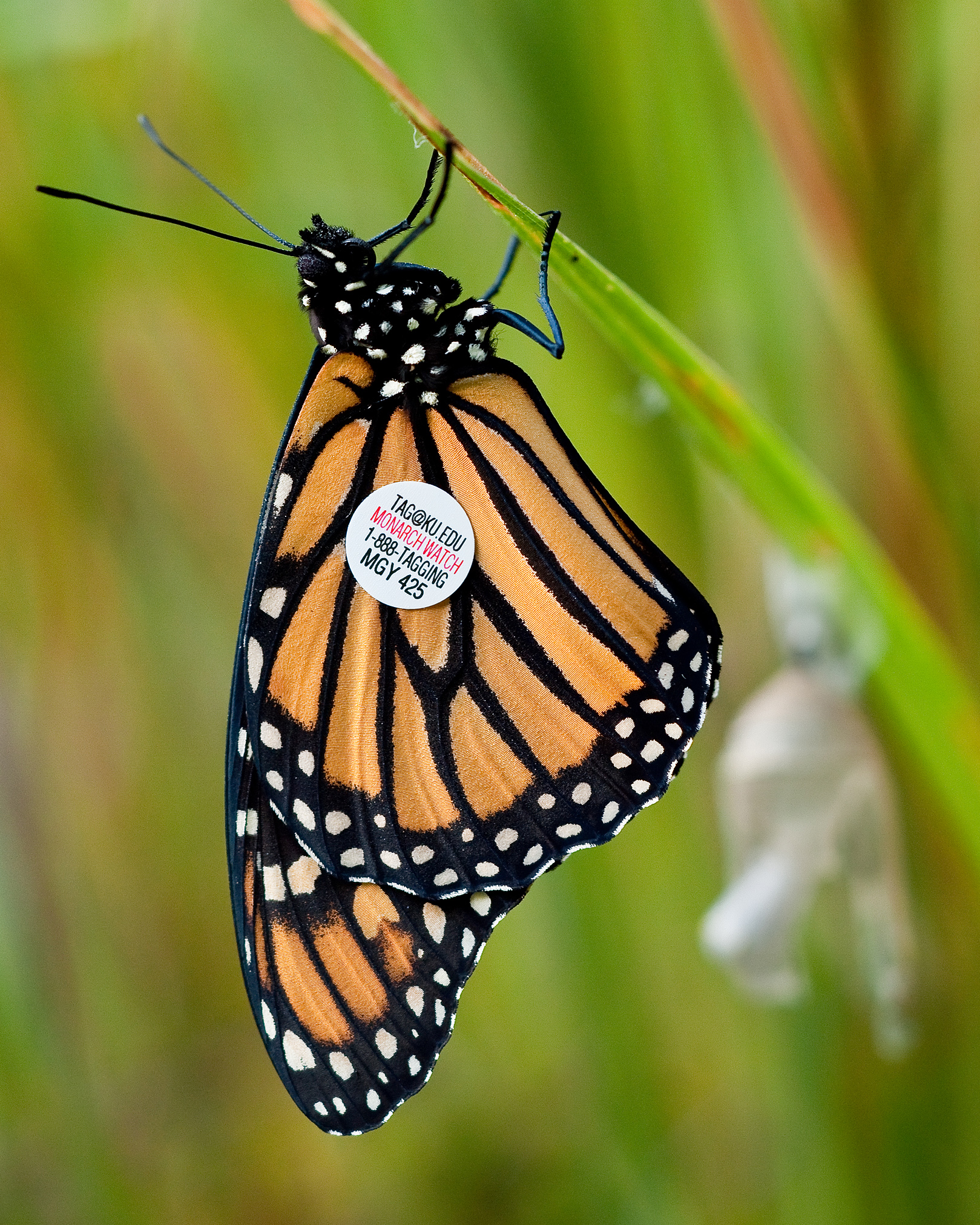A close-up photograph captures the vibrant details of a Monarch butterfly. The butterfly, predominantly orange with contrasting black stripes, clings delicately to a green plant stem. Its wingtips and body are marked with a striking pattern of black interspersed with white dots. The background is a soft, blurry green, drawing attention to the subject. A small circular tag on one of the butterfly’s wings bears the text “tag at ku.edu” in black letters and “Monarch Watch” in red letters, indicating it is part of a tracking program. Additionally, it displays the identification code "1-888-TAGGING-MGY-425" in black letters.